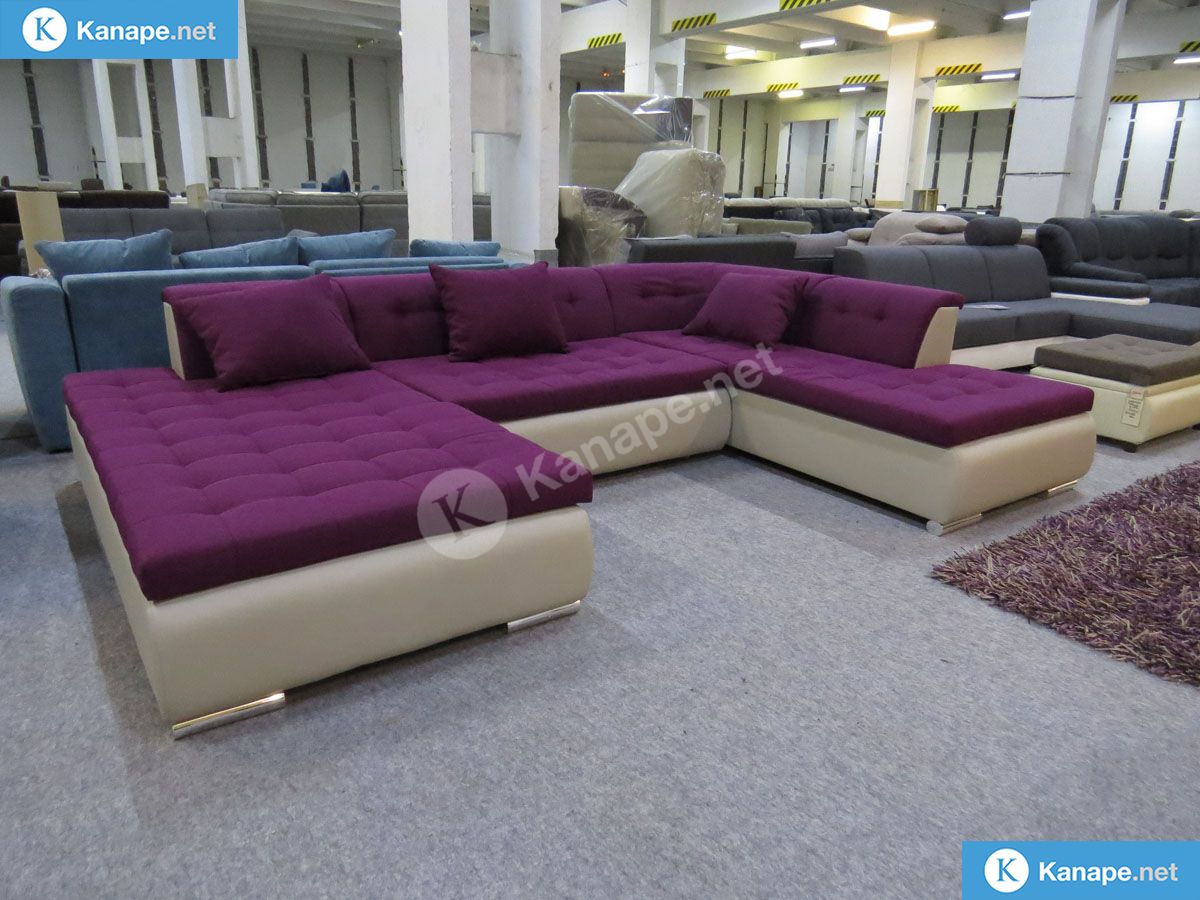This is an image from a furniture showroom identified as Canape, or canopy.net (K-A-N-A-P-E.net). Dominating the foreground is a large, modular U-shaped sectional sofa, composed of three pieces joined together. The sofa features a light gray vinyl base with silver feet, complemented by deep purple cushions and pillows. A striking purple and gray throw rug sits nearby, accentuating the sofa's modern design.

The showroom's plain gray carpet underpins a variety of modern-looking furniture. In the background, numerous other couches and futons in various colors, including pink, blue, and gray, are displayed, with some pieces still wrapped in plastic. The space is fluorescently lit, adding a bright, clean ambiance to the extensive display of contemporary seating options. The name of the store, canape.net, is visibly marked in both the upper left and lower right corners of the store.